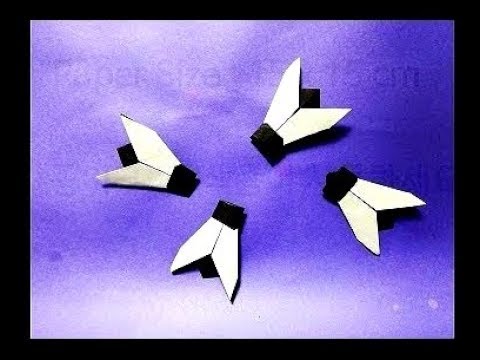The artwork is a computer-generated image encased in a wide, black vertical frame. It features a purple background that transitions from dark purple at the top to almost white at the bottom, evoking the impression of a cloudy, purple-tinted sky. There are four distinct objects on this purple gradient, each resembling a paper airplane with white wings and black heads and tails, suggesting an insect-like form with the angularity of a jet aircraft. These paper airplane-like designs form an upside-down V-shape, connected by a black dotted line with a black square at the bottom. Each airplane is positioned at different angles: one descends from the center left, another rises from the bottom, the third one dives from the top right, and the fourth ascends from the bottom right. The overall effect is a blend of geometric precision and artistic abstraction, creating a visually complex and intriguing composition.